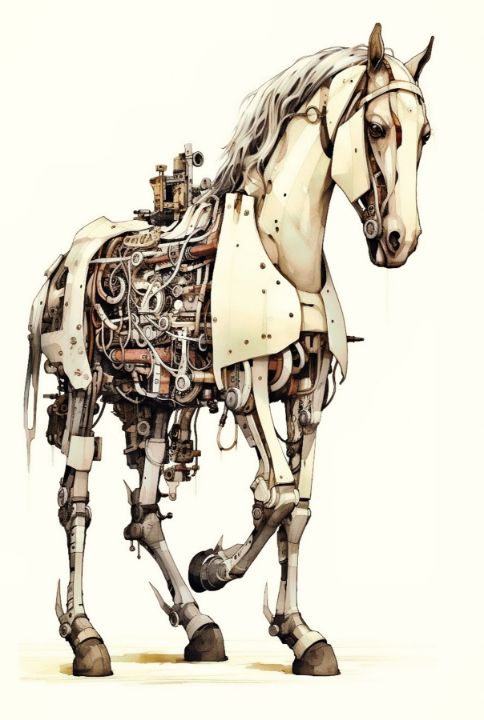The illustration depicts a galloping mechanical horse, viewed at an angle, with dynamic detail in its exposed inner mechanisms. The horse's midsection and legs reveal an intricate array of wires, pistons, and gears, with mechanical hinges visible in the limbs, which are actively moving. Its right front leg is raised, simulating a mid-trot or gallop, while the other hooves are grounded, emphasizing motion. The horse's face is covered with artificial skin, giving it naturalistic features such as ears, a mane, and a stoic expression, although parts of its mouth expose animatronic components. The design includes a thin tail and cream-colored artificial skin covering parts of its chest and neck. Additionally, a cluster of mechanical devices is perched on its back, where a person would typically sit. The background is stark white, complementing the pale, muted tones of the horse's exterior, which includes shades of white, gray, and light brown.